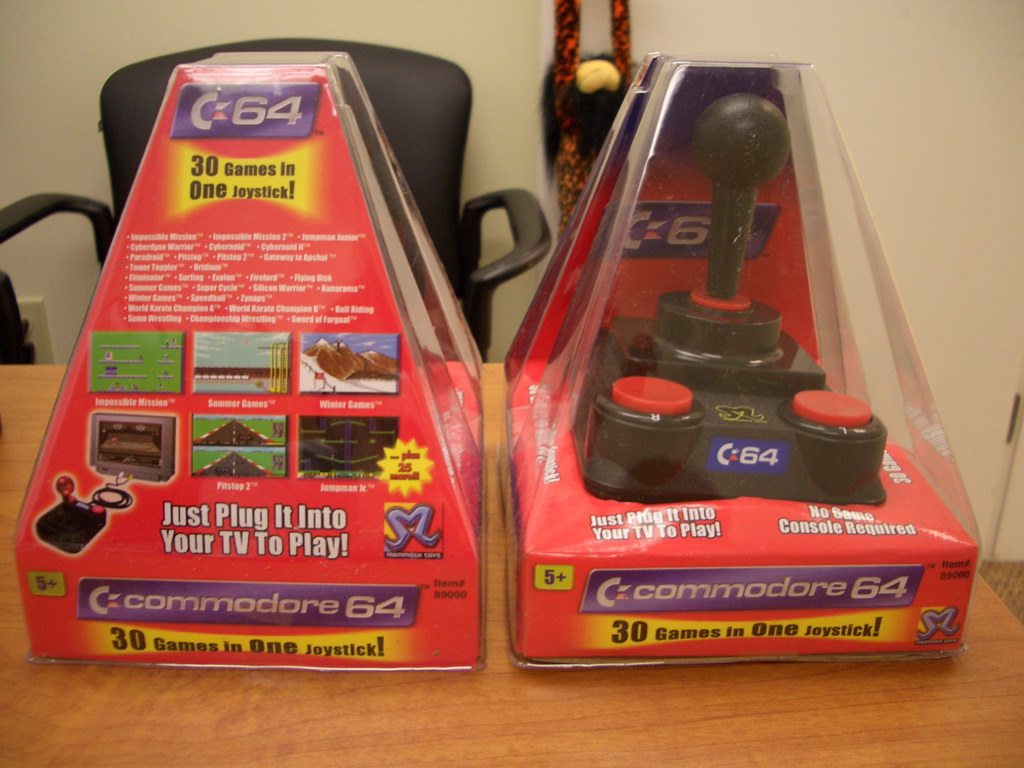This photograph captures two identical models of a retro gaming joystick, known as the Commodore 64 30 Games in One Joystick, displayed in their clear, pyramid-shaped packaging. The packaging itself features a vibrant design with a purple banner sporting white text that reads "Commodore 64," and a yellow banner with black text announcing "30 games in one joystick." The joysticks are predominantly black with large, red circular buttons and a movable lever offering 360-degree control.

Both the front and back views of the packaging are visible, showcasing detailed information. The front side emphasizes the product’s plug-and-play nature, indicating no console is required, and targets users aged 5 and up. The back side lists all the included games and features various screenshots.

The scene is set in what appears to be an office, evidenced by a brown wooden table and a black, fabric office chair in the background. A quirky, monkey-like toy hangs on the wall, adding to the informal atmosphere. The imagery and setting collectively underscore the nostalgic appeal and user-friendly attributes of the product.